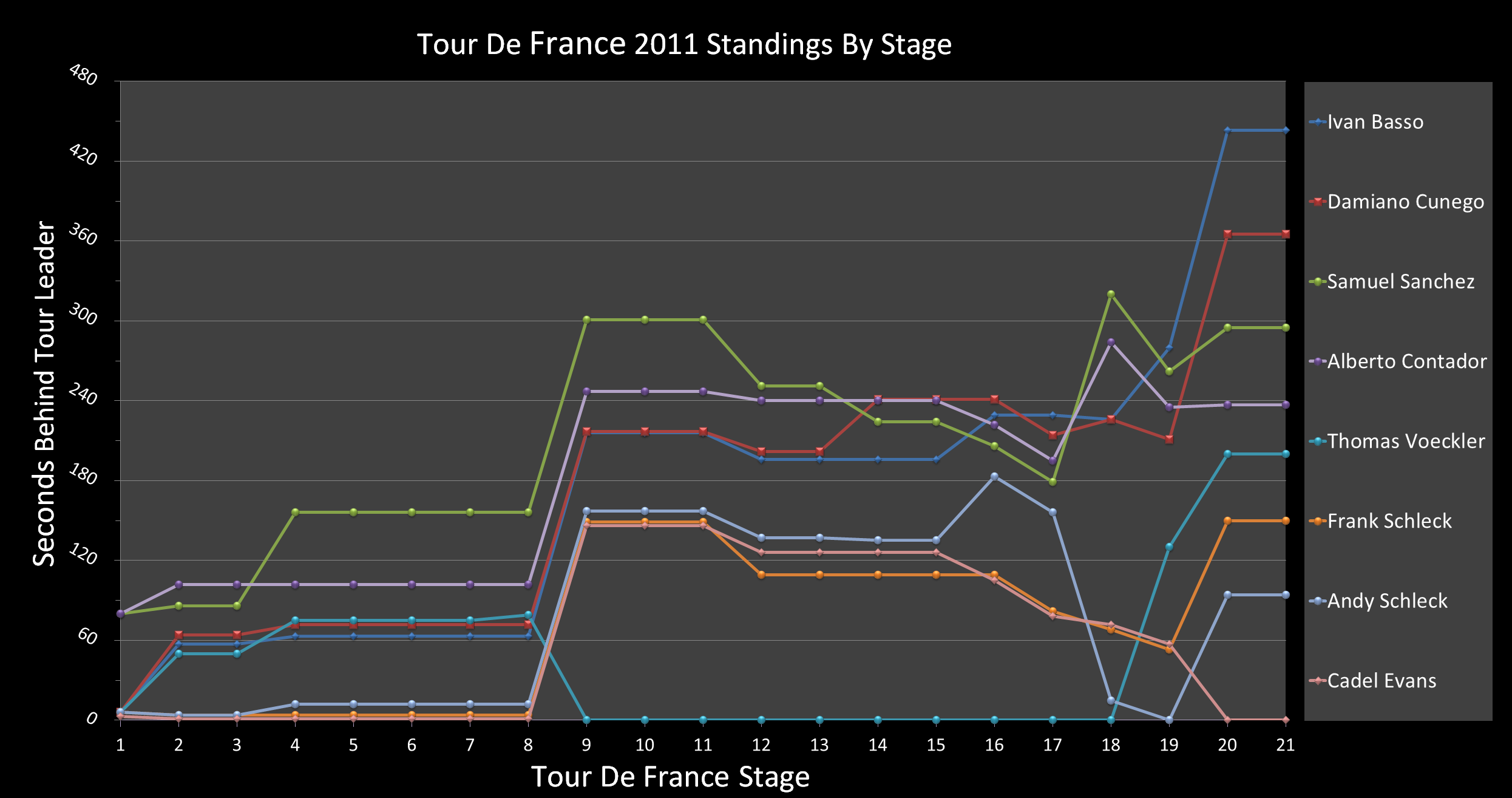This image displays a bar graph on a solid black background, detailing the standings of various participants in the 2011 Tour de France over 21 stages. The vertical axis on the left is labeled “Seconds Behind Tour Leader” in white text, with a range from 0 to 480 seconds. Each stage of the Tour de France is represented horizontally along the bottom, numbered from 1 to 21.

On the right side of the graph, a legend assigns a unique color to each cyclist’s bar line:
- **Blue**: Ivan Basso
- **Red**: Damiano Cunego
- **Green**: Samuel Sanchez
- **Purple**: Alberto Contador
- **Light Blue**: Thomas Voeckler
- **Orange**: Frank Schleck
- **Pink**: Cadel Evans

The colored bars advance through the horizontal stages, intersecting as the participants change positions throughout the race. Ivan Basso's blue, Damiano Cunego’s red, Samuel Sanchez’s green, and others, are meticulously tracked, visually representing their fluctuating distances behind the tour leader. The final standings appear to align with the order in which these cyclists are listed in the legend, illustrating their overall performance by the conclusion of the 21 stages.